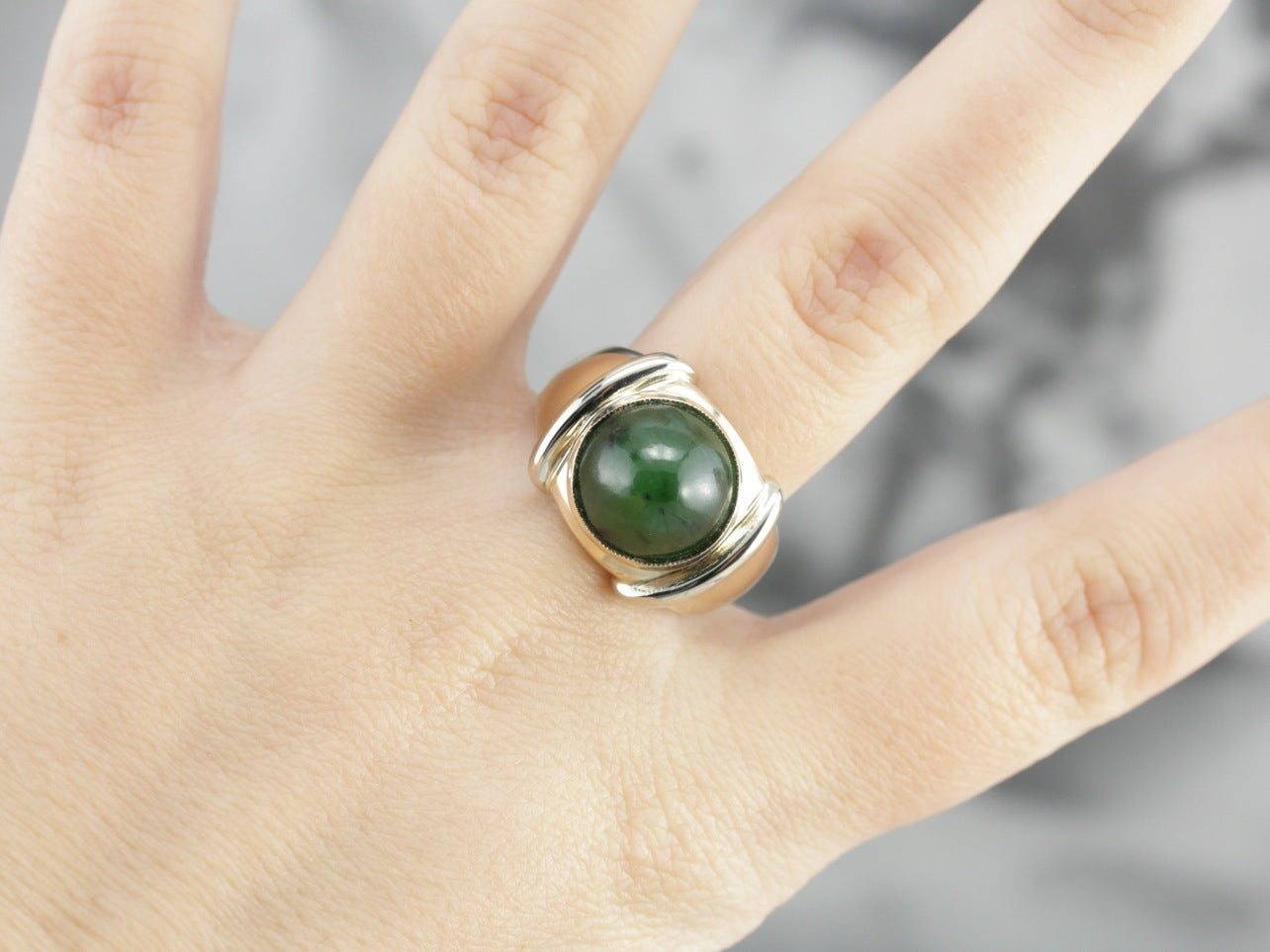In this bright, well-lit image featuring a blurred white and grey background, the focus is on the right hand of a young person with light, white skin. The hand is positioned so that the thumb is not visible, showcasing the middle section of the fingers and part of the back of the hand. Notably, on the middle finger, there is a shiny, thick, golden ring adorned with a large, dark green, glassy gem. The gem, roughly the size of a marble or the black part of an eye, prominently protrudes from the band. The golden band itself has a round, bubbly appearance with ridges on both sides, adding texture to its otherwise smooth surface.